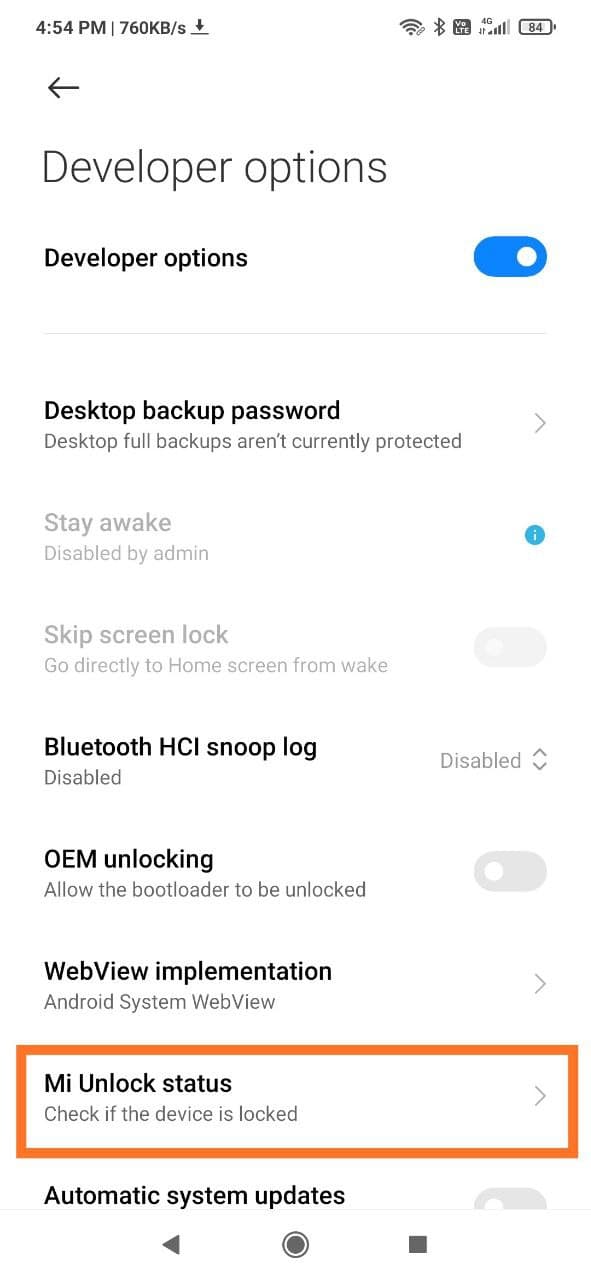The image is a screenshot of a cell phone displaying the Developer Options settings. In the top left corner, the time reads 4:54 PM. Adjacent to the time, a file is currently downloading. Moving to the right, there are icons for Wi-Fi, Bluetooth, and the battery percentage.

Below these status icons, a left-pointing arrow indicates a back option. Following this, the text "Developer Options" appears twice: once in regular font and again below in smaller, bolder black text. To the right of this second "Developer Options" text is a blue toggle button indicating that Developer Options are enabled.

Below the Developer Options header, several settings and their states are listed. It starts with "Desktop backup password" and a note that desktop full backups are not currently protected. Next, there are options labeled "Stay awake," "Skip screen lock," and "Go directly to home screen from wake," with a note under "Stay awake" that it is disabled by the administrator.

Further down, there is a "Bluetooth HCI snoop log," which is disabled, and "OEM unlocking" with the description "Allow the bootloader to be unlocked," currently turned off. Following this is "WebView implementation" set to "Android System WebView." An orange rectangle highlights the "MI Unlock Status," which advises users to check if their device is locked. Finally, "Automatic system updates" is shown without any additional note.

At the bottom of the screen are three navigation icons: a dark gray triangle pointing left, a circle in the center, and a square to the right.